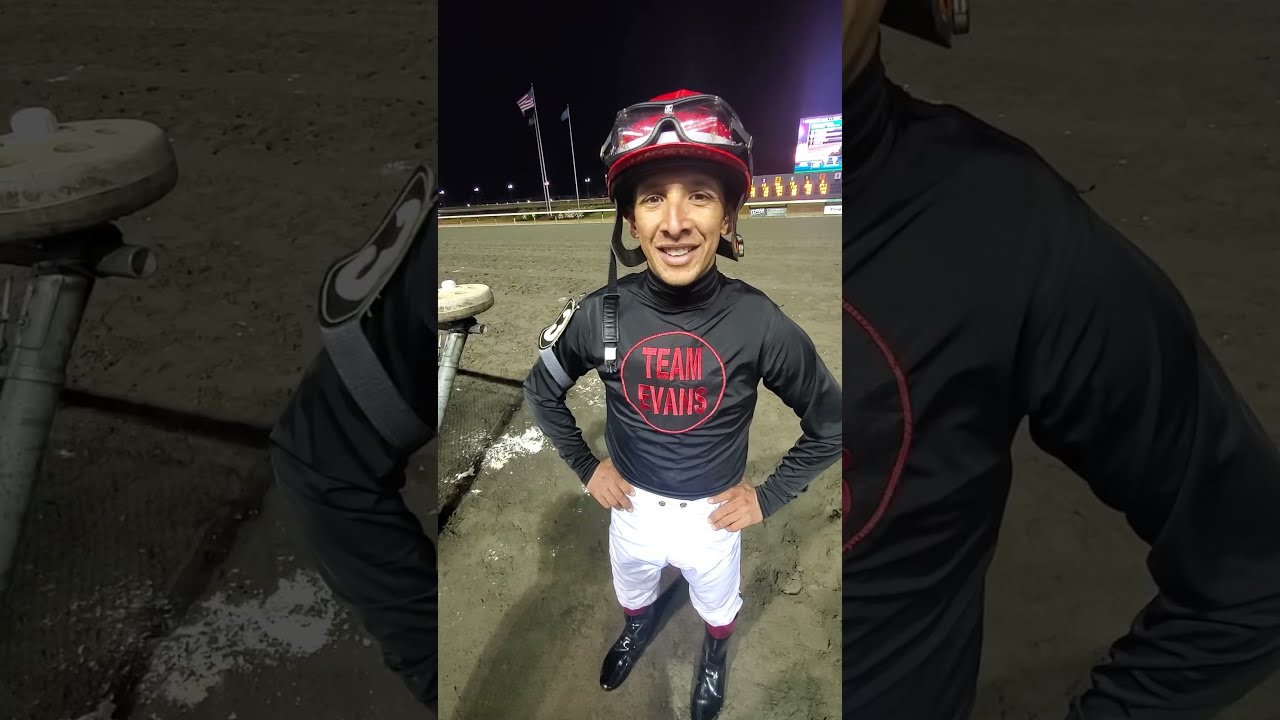This image captures a jockey standing outdoors on a horse racing track at night. The central figure, photographed vertically on a phone, is overlaid against a horizontally oriented backdrop. The jockey wears distinct attire: a black, long-sleeved shirt with a red circle featuring "Team Evans" in red text, white pants, red socks, and black boots. He sports a red helmet with black goggles perched on top, and a microphone at the end of the helmet. His posture is confident, with hands placed on his hips and a smile directed at the camera.

The background features a dirt track, characterized by its brown and gray hues. Two tall white flagpoles with American flags are visible to the left, waving against the dark night sky. A fence post and a large, distant screen with blue and pink illumination are discernible on the right. The left and right sides of the overall image are shadowy, zoomed-in sections of the central photograph, adding depth to the composition. The scene is subtly enriched by the shadow of the photographer, visible in the bottom left corner.